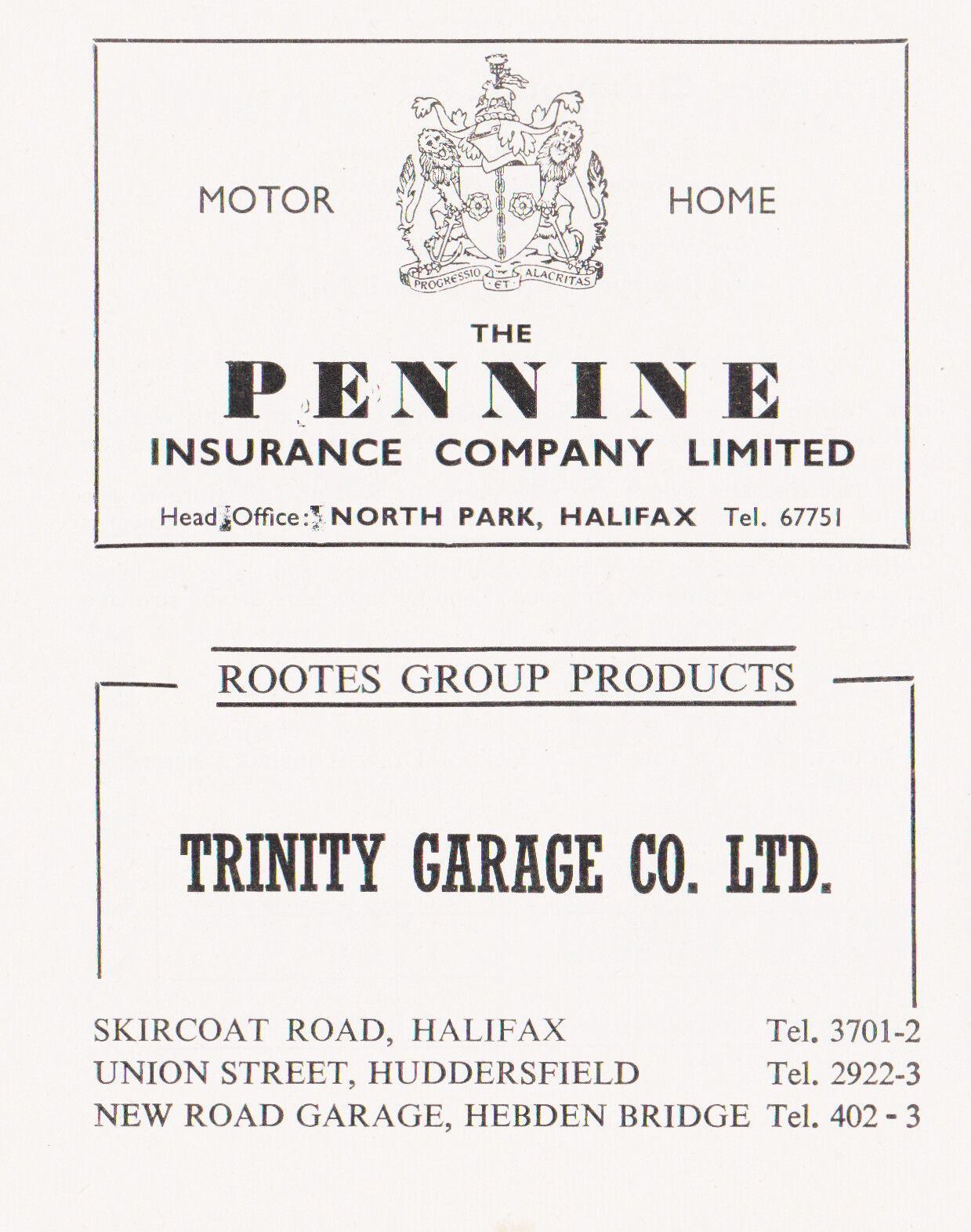This image is an advertisement on a white background. At the top, there is a black-outlined square featuring the word "Motorhome" alongside a regal emblem. Below this, in bold lettering, it reads "The Pennine Insurance Company Limited, Head Office, North Park, Halifax, TEL. 67751." Following this, another black square contains the text "Roots Group Products." Beneath this, in a bolder font, it states "Trinity Garage Company Limited." Further down, smaller text indicates multiple locations with their respective details: "Skirkote Road, Halifax, TEL. 3701-2," "Union Street, Huddersfield, TEL. 2922-3," and "New Road Garage, Hebden Bridge, TEL. 402-3." The font throughout the ad is black, contrasting against the white background.